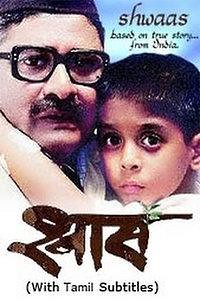The image is an advertisement for a movie titled "Shwas," based on a true story from India. In the foreground, there is a man with black-rimmed glasses, a mustache, and a concerned expression on his face. He is holding a little boy with black hair and dark eyes, who also looks frightened and has his arms wrapped around the man's neck. The background of the image is blue, resembling the sky, which enhances the visual appeal. There is text underneath the picture, with some writing in a foreign language in brown, and a caption in parentheses that reads "(with Tamil subtitles)." At the top right corner of the image, the title "Shwas" is prominently displayed. This appears to be the front cover of a CD or a promotional poster for the movie.